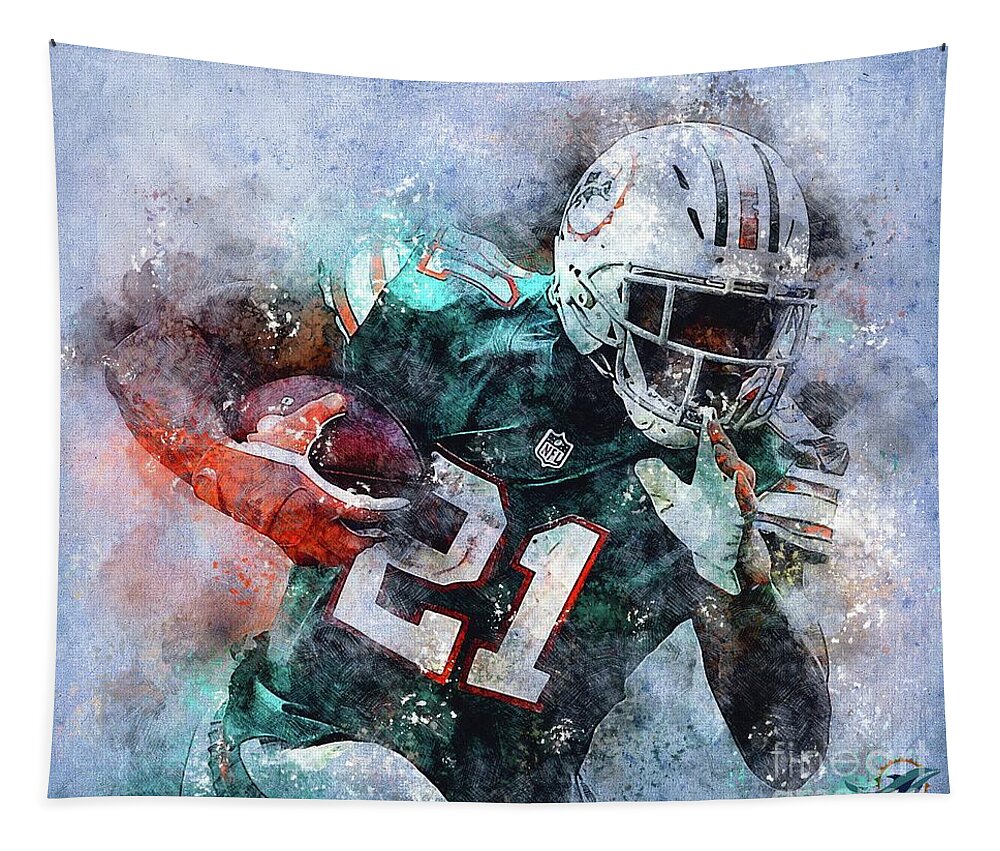The image depicts a Miami Dolphins football player running with a football under his right arm, shown from the waist up. The player, an African-American man, is wearing an unmistakeable Miami Dolphins uniform: a green jersey with the number 21 in white on his chest, and a white helmet adorned with the team's emblem and stripes across the top. He is also seen sporting orange gloves. The background of the image features smudges and splatters of red, black, and gray paint, creating a foggy, cloud-like effect that contrasts with the detailed center of the piece. The tapestry, attached to a white wall with small tacks in the upper corners, displays the Fine Art watermark and a Miami Dolphins logo in the bottom right corner. The entire scene is presented in a realistic yet graffitied style, with blurred paint adding a dynamic, artistic touch to the depiction.